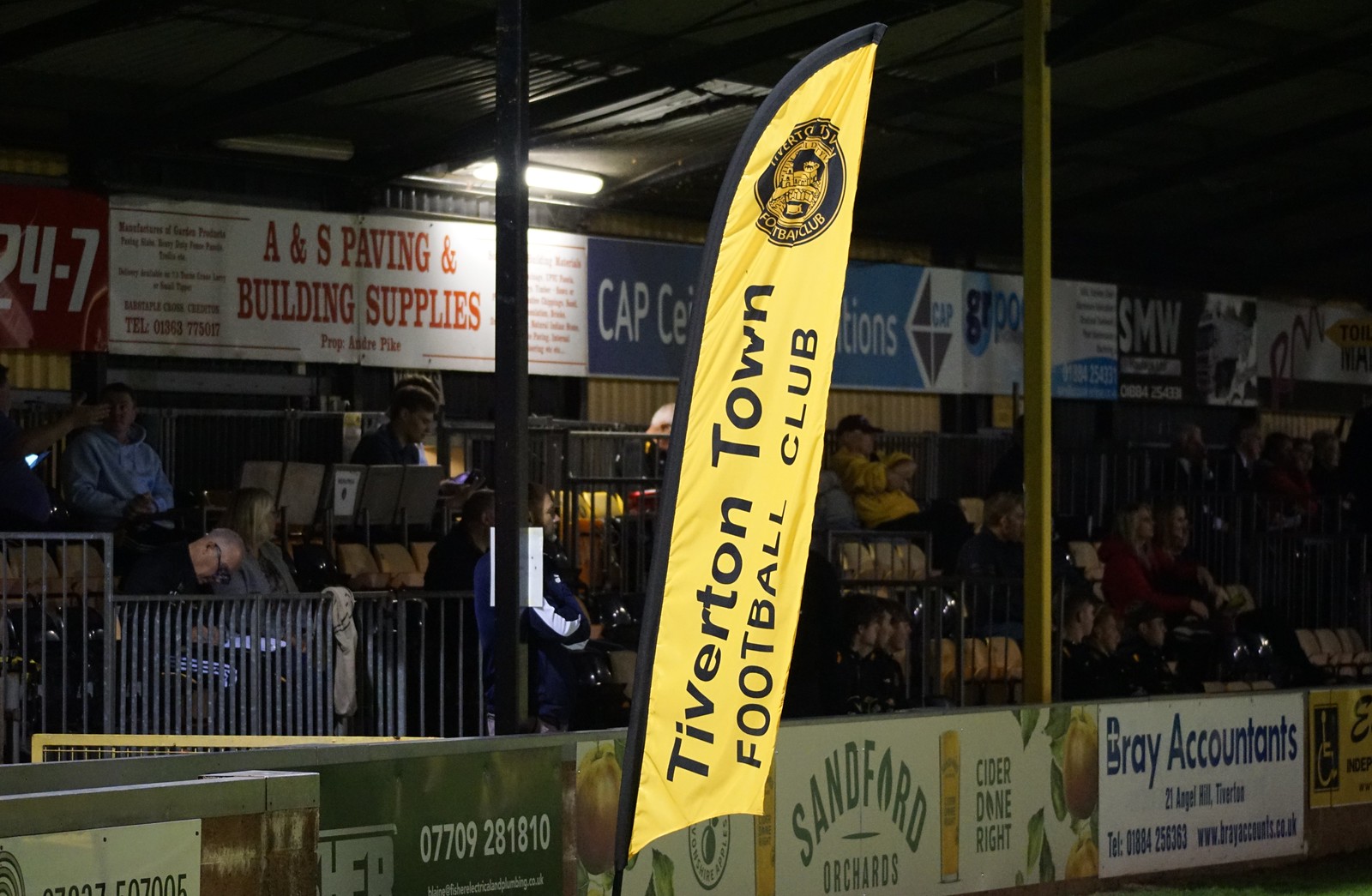In this detailed image of a sports arena, the focal point is the tall, centrally positioned yellow banner that proudly states "Tiverton Town Football Club" in black text, along with a circular logo at the top. Directly below this banner is a seating area filled with spectators. The audience area is framed by a lower section of fencing adorned with multiple sponsor banners, which include ads for companies such as Sanford Orchards, Bray Accountants, and ANS Paving and Building Supplies.

The arena, captured at night, appears to be indoors. Overhead, a single light fixture hangs in the center of the ceiling, casting a glow on the audience and banners below. Multiple advertisements are scattered throughout the image, both beneath and above the seated spectators, displaying various company names and logos, such as those featuring fruit images and contact information.

The overall color palette of the scene includes gray, white, black, green, yellow, blue, red, and orange, highlighting the vibrant and busy atmosphere of the venue. The environment provides a glimpse into the sponsorship-laden setting typical of a sports event, even though the playing field itself is not visible.